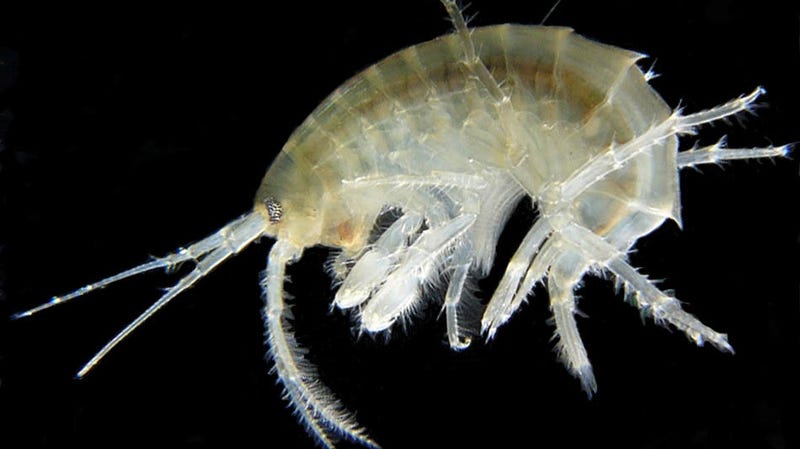This medium-quality photograph, approximately eight to nine inches across by five inches tall, features a striking depiction of a translucent shrimp, set against a stark black background. The shrimp is oriented on its side, with its head to the left and its body curving slightly as its tail tucks towards its middle. Through its semi-transparent shell, the intricate internal anatomy, including a spine-like structure, is distinctly visible, creating a high-contrast, almost artistic effect. The shrimp’s body, predominantly white with hints of potential browning or yellowing, reveals detailed features such as a pair of black eyes dotted with white, and four prominent antennas—two extending forward and two dangling covered with fine hairs emerging from its mouth. The image's high-contrast nature between the shrimp’s vivid details and the dark backdrop lends it an x-ray-like, jarring quality, emphasizing the shrimp's delicate and intricate structure.